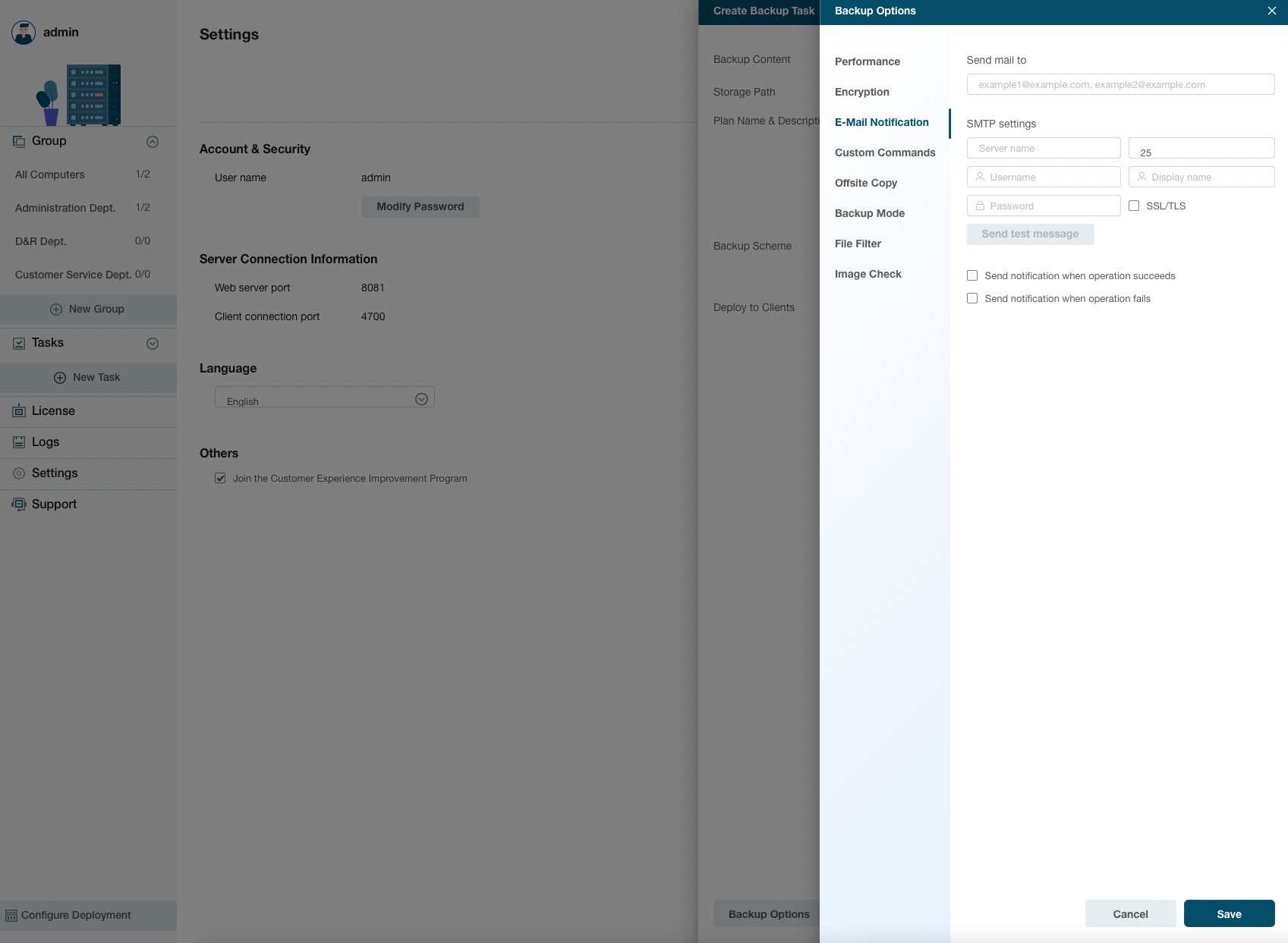This digital interface image features an administrative settings panel. In the upper portion, there is a small, animated male character icon situated next to the "Admin" label. Adjacent to this is a digital plant and a building icon. 

Below these, the interface displays several groups and departments such as "Group 1/2," "All Computers," "Administration Department," "DNR Department 0/0," and "Customer Service Department 0-0." Additionally, there are options to create a "New Group," "Task," or "New Task."

Located towards the bottom are links labeled "License," "Logs," "Settings," and "Support," providing quick access to various resources. There is also a section for "Account and Security," showing the username "Admin" along with a button to modify the password. 

Furthermore, server connection information is displayed, indicating the web server port as 8081 and client connection port as 4700, with the language set to English. This detailed layout ensures that various administrative functions and settings are easily accessible.